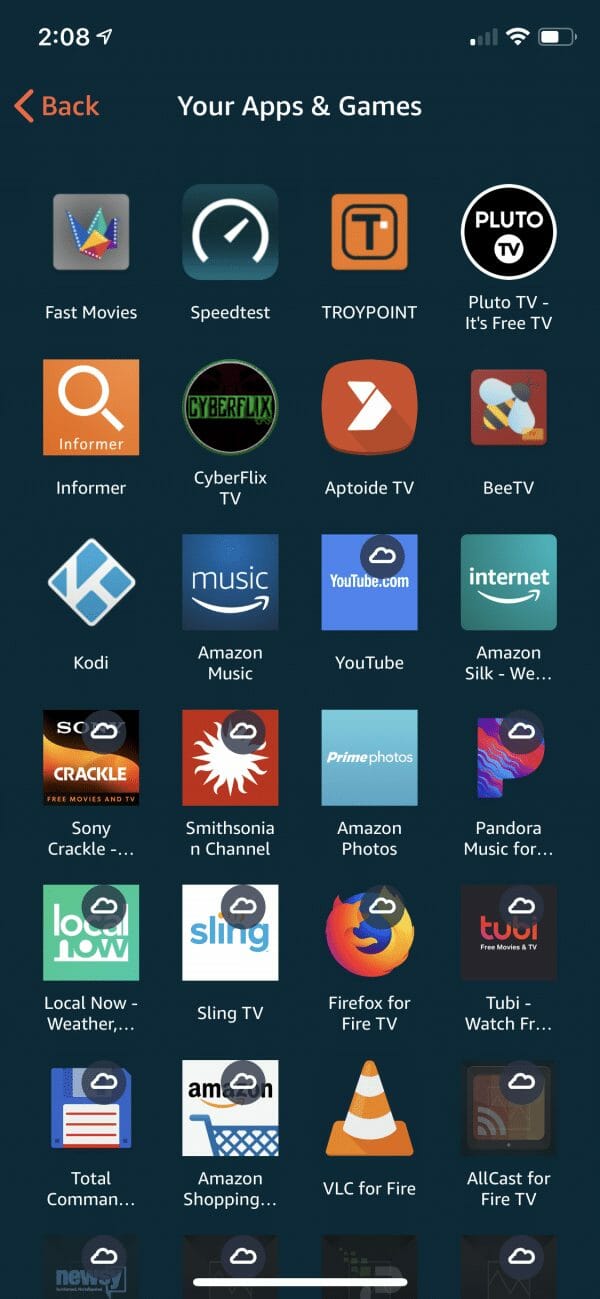Screenshot Description:

This is a detailed screenshot from a smartphone with a black background. In the top-left corner, the time is displayed in white numerals as "2:08." To the right of the time, there is a battery icon that indicates approximately 75% charge.

Below the status bar, a left-pointing arrow accompanies the word "Back." In the center, the header displays "Your Apps & Games" in white text.

The apps are organized in several horizontal rows:

1. The first row includes Fast Movies, Speed Test, TROYPOINT, and Pluto TV (noted as free TV).
2. The second row lists Informer, CyberFlix TV, Aptoide TV, and VTV.
3. The third row features Kodi (repeated twice), Amazon Music, YouTube, and Amazon Silk Browser.
4. The fourth row consists of Sony Crackle, Smithsonian Channel, Amazon Photos, and Pandora Music.
5. The fifth row displays Local Now Weather, Sling TV, Firefox for Fire TV, and Tubi.
6. The sixth row includes Total Commander, Amazon Shopping, VLC for Fire, and Allcast for Fire TV.

The entire screen is framed at the bottom by a thin white line.